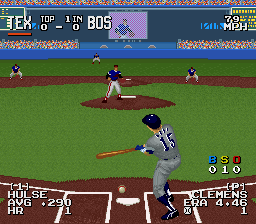This is an image of a pixel-art baseball video game, capturing an intense moment of gameplay. The scene is set in a stadium with detailed, albeit pixelated, digital crowds filling the stands against a blue back wall. Central to the image is a baseball diamond with a vividly brown pitcher's mound. The pitcher, garbed in a blue shirt, white pants, and a cap, stands poised on the mound. Defensively positioned are an outfielder, a second baseman, and a midfielder.

In the forefront, closest to the viewer, stands the batter inside the designated batter's box, identifiable by the home plate at his feet. The batter, wearing a gray uniform adorned with the number 15 and a dark cap, is right-handed, with his bat nearly parallel to the ground, a ball clearly visible over the plate underneath him. Above and beside the gameplay, the screen displays various in-game statistics, including text in the top left reading "zero, one, in, zero, and boss," as well as player information featuring names such as Clemens. Additionally, the bottom of the screen includes data and numerical values, with distinctively colored indicators (blue, yellow, and red) marked "BSO" and the number "010."